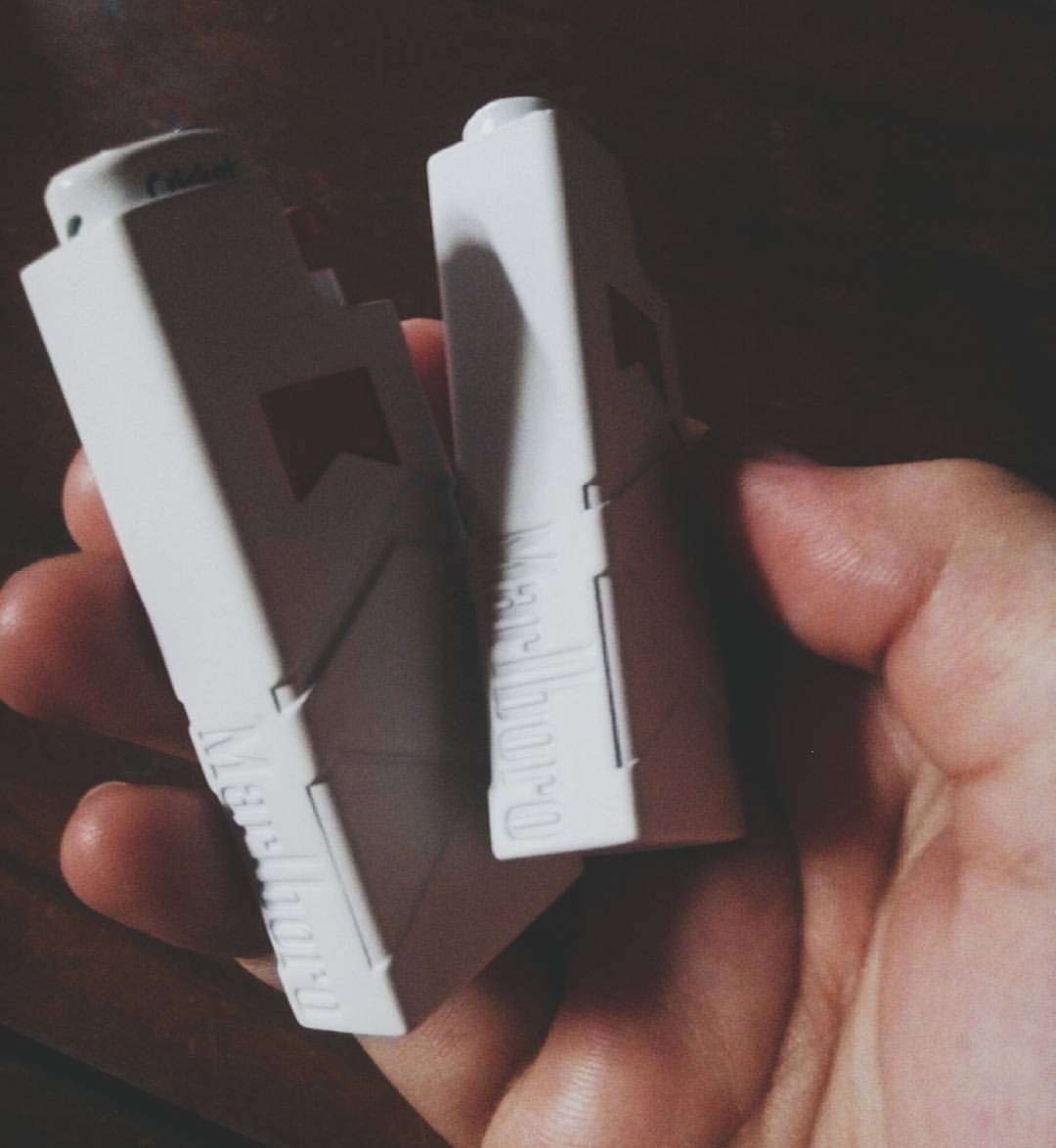The image is a grainy, low-resolution color photo featuring a man's right hand with visible pinky, ring, and middle fingers, as well as parts of the pointer finger and thumb, with a slight glare of light obscuring part of the photo. The hand, against a completely black background, is holding two identical white plastic flasks. Each flask is rectangular with the word "Marlboro" imprinted on the side. The flasks appear to be cigarette cases with a clip or flap on the front for opening, and a circular housing at the top, possibly intended for lighters. The exact wording on one of the flasks is partially obscured by the glare.